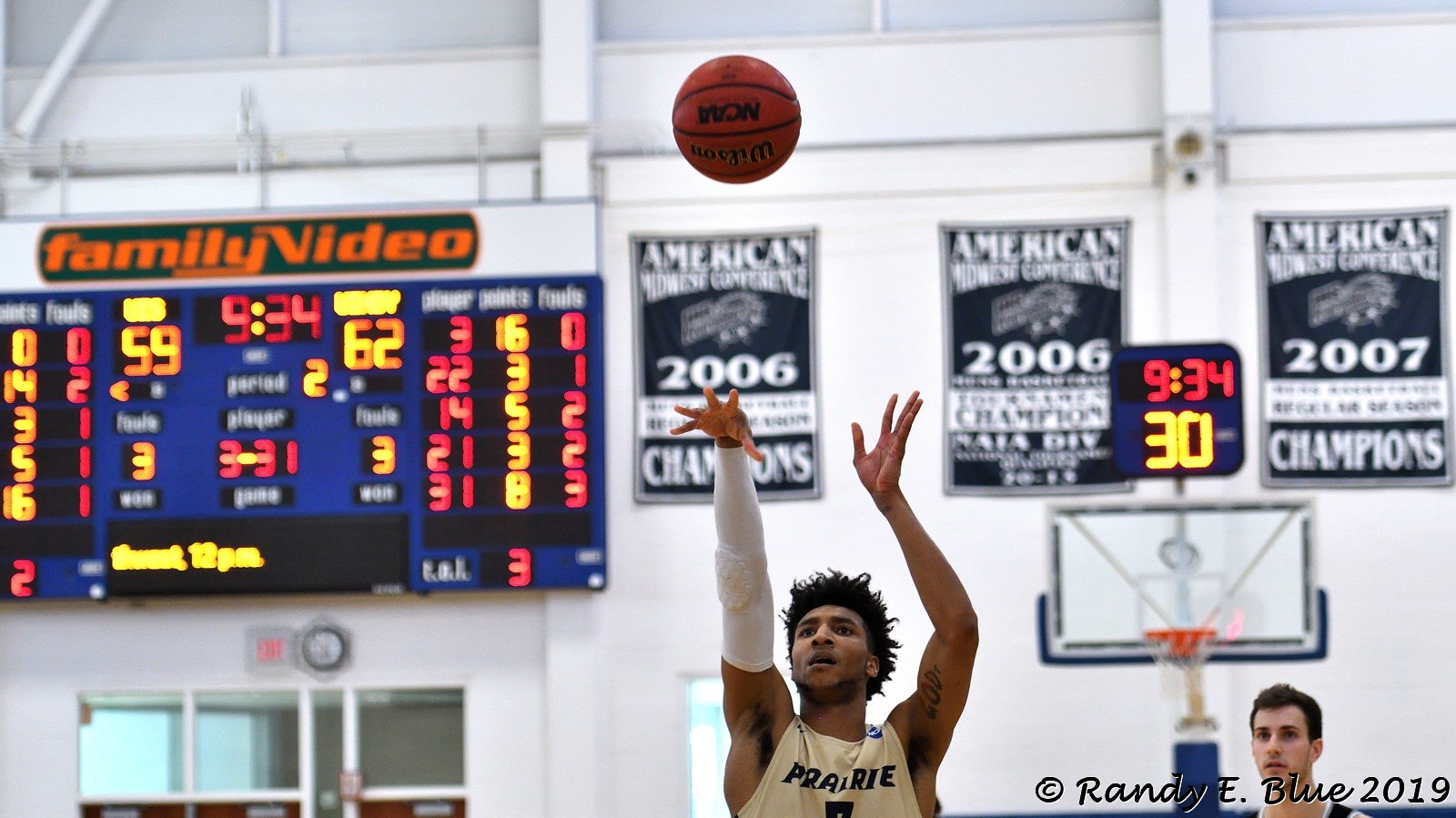In this detailed sports photograph of a high school basketball game, the shot captures the intense action of a player in mid-shot. The player, an African-American male, is prominently featured from the chest up, wearing a white jersey with blue accents that reads "Prairie" and a white shooting sleeve on his right arm. He is releasing a Wilson NCAA basketball with his right hand, with the ball already a few feet out from his fingertips, crested above his head. His left arm is extended slightly to the side, having just guided the ball. Opposite him, a defender in a blue jersey and with brown hair is partially visible in the lower right corner, looking on.

Dominating the top left of the frame is a large blue scoreboard underneath a "Family Video" sign, showing a score of 59-62 in the second period with 9:34 remaining and 30 seconds left on the shot clock. Foul counts are displayed as three for each team, with illuminated player rosters denoting points and fouls in red and yellow digits. The background features a stark white wall adorned with several black-and-white championship banners, including those marking "American Conference 2006 Champions" and "2007 Division Champions." Also visible is the opposite basket, providing depth to the scene. In the lower right-hand corner, the image is credited with "Randy E. Blue, 2019" marked alongside a copyright symbol.